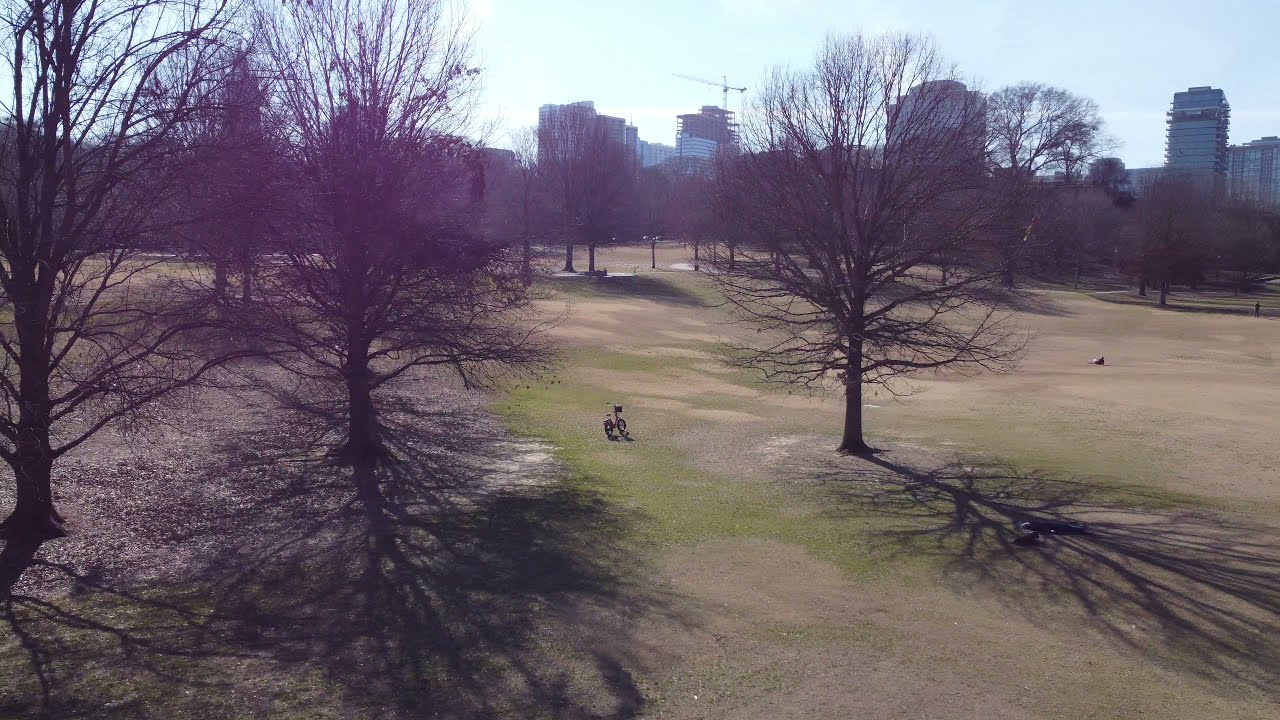This image captures a park nestled within a city, evident from the backdrop of five tall skyscrapers. It's a bright, sunny day, and the sky is a clear light blue peppered with a few clouds. The large grassy field dominating the scene is a mix of green in the center and a faded yellow-brown toward the edges. Scattered across the park are multiple leafless trees casting distinct shadows on the ground, suggesting it's wintertime. 

On the left, beneath two of these trees, there's a grayish area that resembles fallen leaves or mulch. A small child’s bicycle is parked under one of the trees on the right side of the image. In the middle of the park, an indistinct figure or object is situated on the grass, adding a focal point to the expansive open space. Additionally, there are a few small concrete areas and possibly a bench or a path that further hint at the park's layout. A crane is visible in the distance, further indicating ongoing urban development nearby.